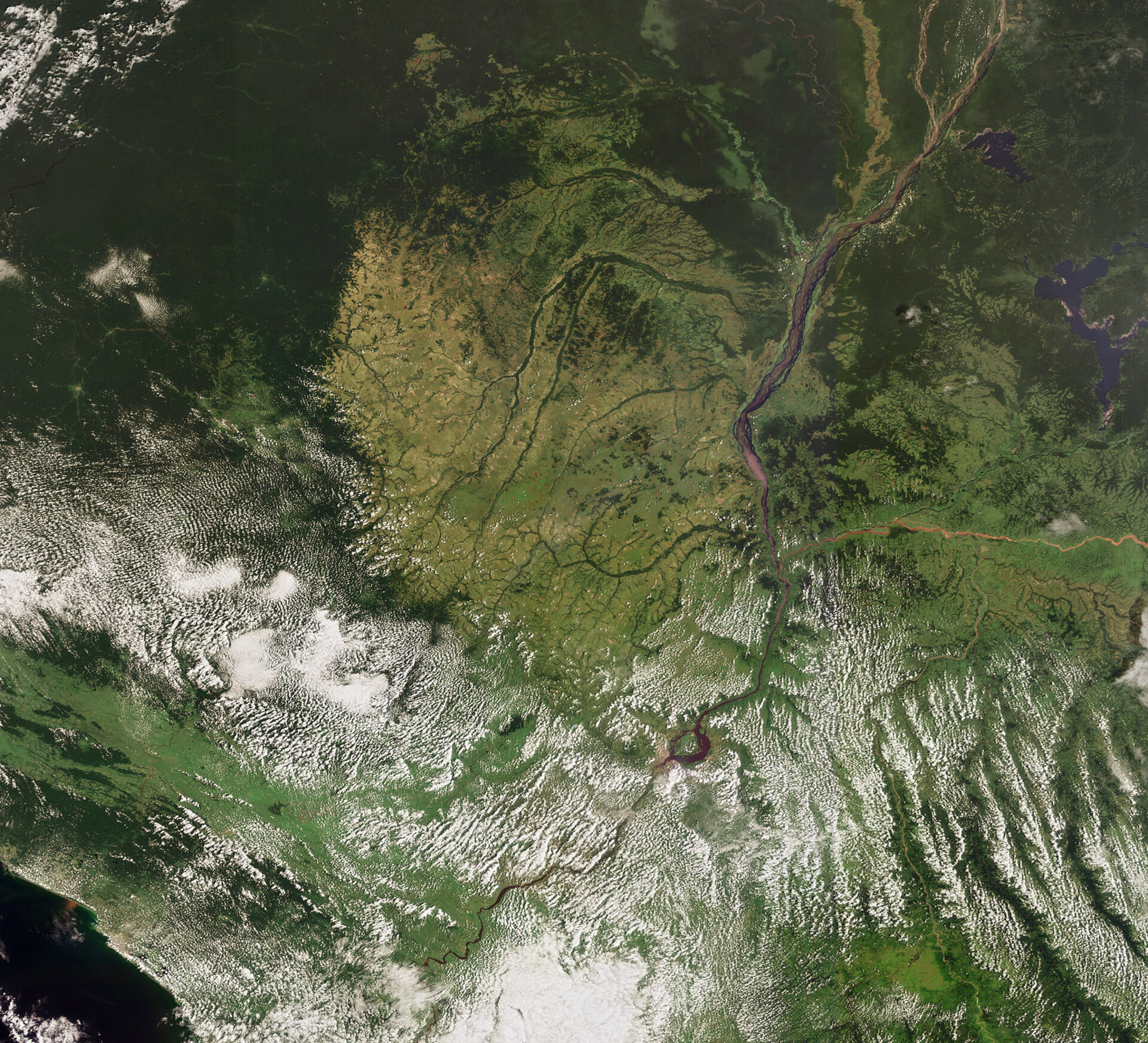This image, resembling a satellite photograph, captures a broad landscape seen from high above, perhaps space. The predominant color is green, indicating fields or forests, interspersed with patches of white that might be snow or clouds. The bottom left corner features a dark patch that likely represents a body of water or the ocean. Ascending from this point, the landscape transitions into areas of green with scattered white elements. Near the upper portion of the image, a thin, long brown feature, possibly a river or tree branch, stretches across the scene. In the upper right corner, a few small, narrow blue regions suggest additional bodies of water, such as lakes or streams. The overall impression is one of a rich, green terrain with complex textures and sporadic water bodies, blending natural elements like water, land, and possibly snow or clouds.